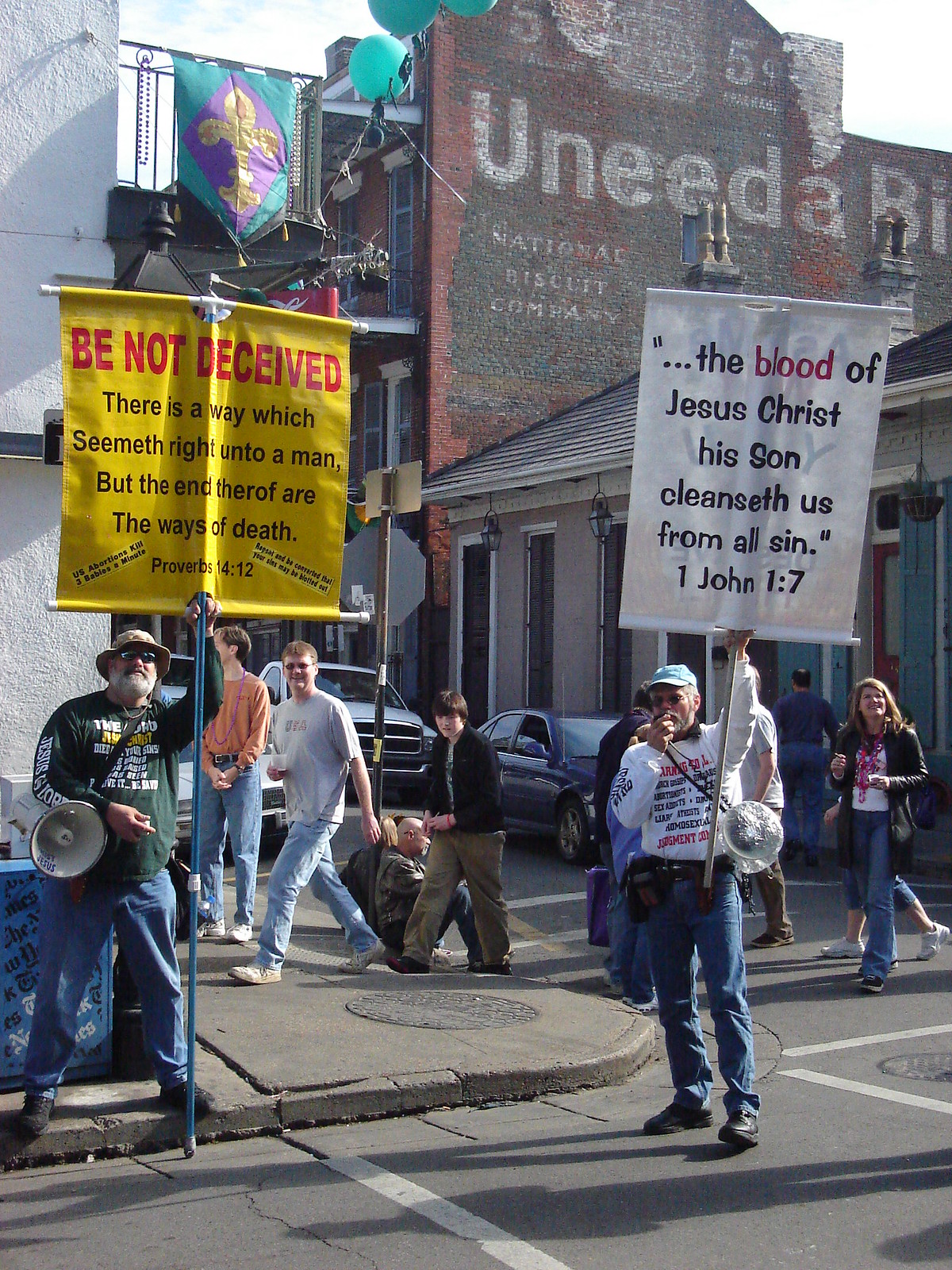This daytime photograph captures a vibrant street corner scene featuring a religious demonstration. On the right, a man in a long-sleeved white t-shirt, adorned with various writings, stands partially on the road holding up a white fabric sign that reads, "The blood of Jesus Christ his son cleanseth us from all sin. 1 John 1:7." To his left, another man wearing a beard, a bucket hat, and a long-sleeved green t-shirt, also covered in writings, stands on the curb. He holds a yellow sign that declares in red letters, "Be not deceived there is a way which seemeth right unto a man, but the end thereof are the ways of death," quoting Proverbs 14:12. This man also has a bullhorn slung over his shoulder. The scene is framed by an old brick building with partial signage that reads "you need a," and across the street is a white building with a balcony, proudly displaying a fleur-de-lis flag. Pedestrians walk by, some crossing the street, seemingly uninterested in the demonstrators' messages.